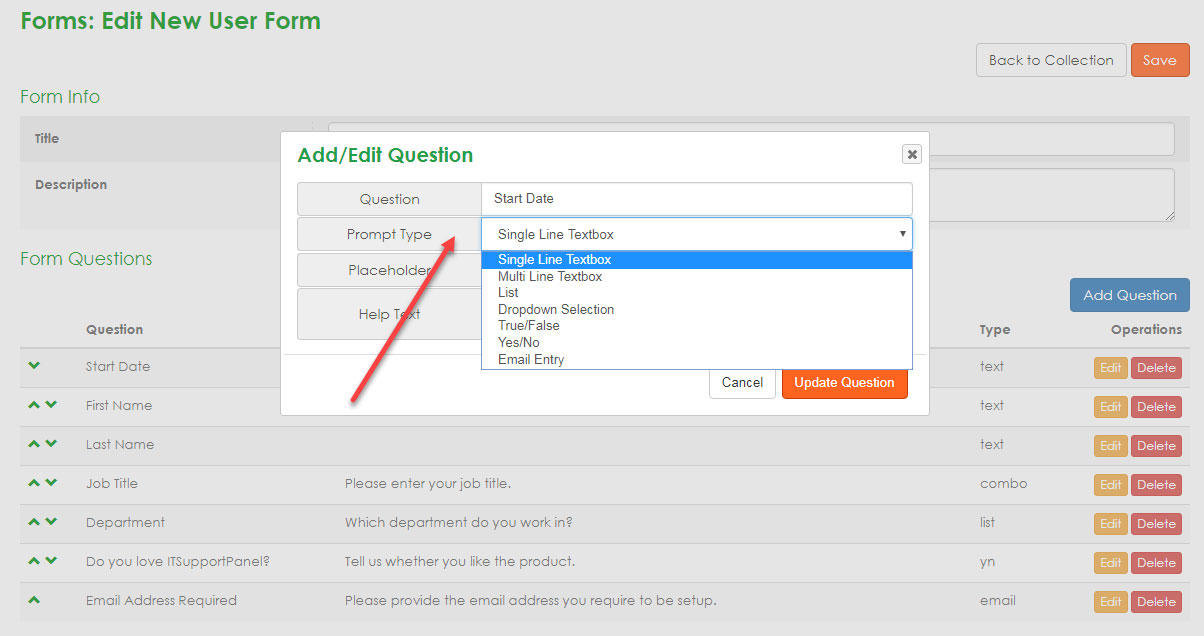The image showcases a user interface for a website's form creation section. The primary header "Forms" is displayed in green, and sections such as "Edit New User Form" and "Form Info" are also highlighted in green. An option labeled "Back to Collection" is situated on the right side of the page. Below this, an orange "Save" button is prominently featured.

A pop-up box partially obscures the screen, featuring options for form customization. This box is labeled "Add/Edit Question." The first field within the pop-up is a question input box, styled in gray. The field for "Start Date" is visible in a white textbox. Following this, there is a prompt type selector, accompanied by a red arrow pointing upward, highlighting the chosen option, "Single Line Text Box." Additional fields labeled "Placeholder" and "Help Text" are present, with "Update Question" and "Cancel" buttons located at the bottom.

Returning to the main website interface, the section titled "Form Questions" lists various fields such as "Start Date," "First Name," "Last Name," "Job Title," "Department," "Do You Love IT," "Support One," and "Email Address." Each of these questions is aligned with an "Edit" button in orange and a "Delete" button in red on the right side.